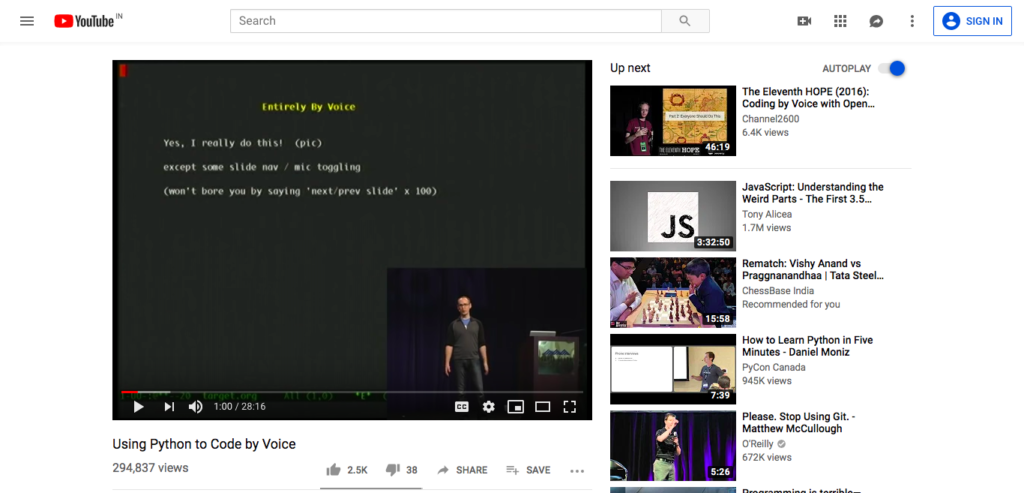**Descriptive Caption:**

"Thank you, Angels. This screenshot is taken from a YouTube video titled 'Using Python to Code by Voice.' In the snapshot, an AI-generated person appears with text overlays in yellow stating 'Entirely by Voice' and 'Yes, I really do this.' Below, in a gray box, additional text notes, 'Except some slide Nov/Mick toggling' and 'Won't bore you by saying next/prev slide times 100.' The user has watched 1 minute of the 28-minute and 16-second video.

On the right side of the screen, the YouTube interface displays various icons: the YouTube logo (a white play button in a red rectangle), a search bar, a 'Create' button (a video plus sign), a grid icon, a notification bell, and a 'Sign In' option featuring a silhouette of a person. Additionally, there is a sidebar on the right displaying a list of suggested videos, with five visible and others cut off."